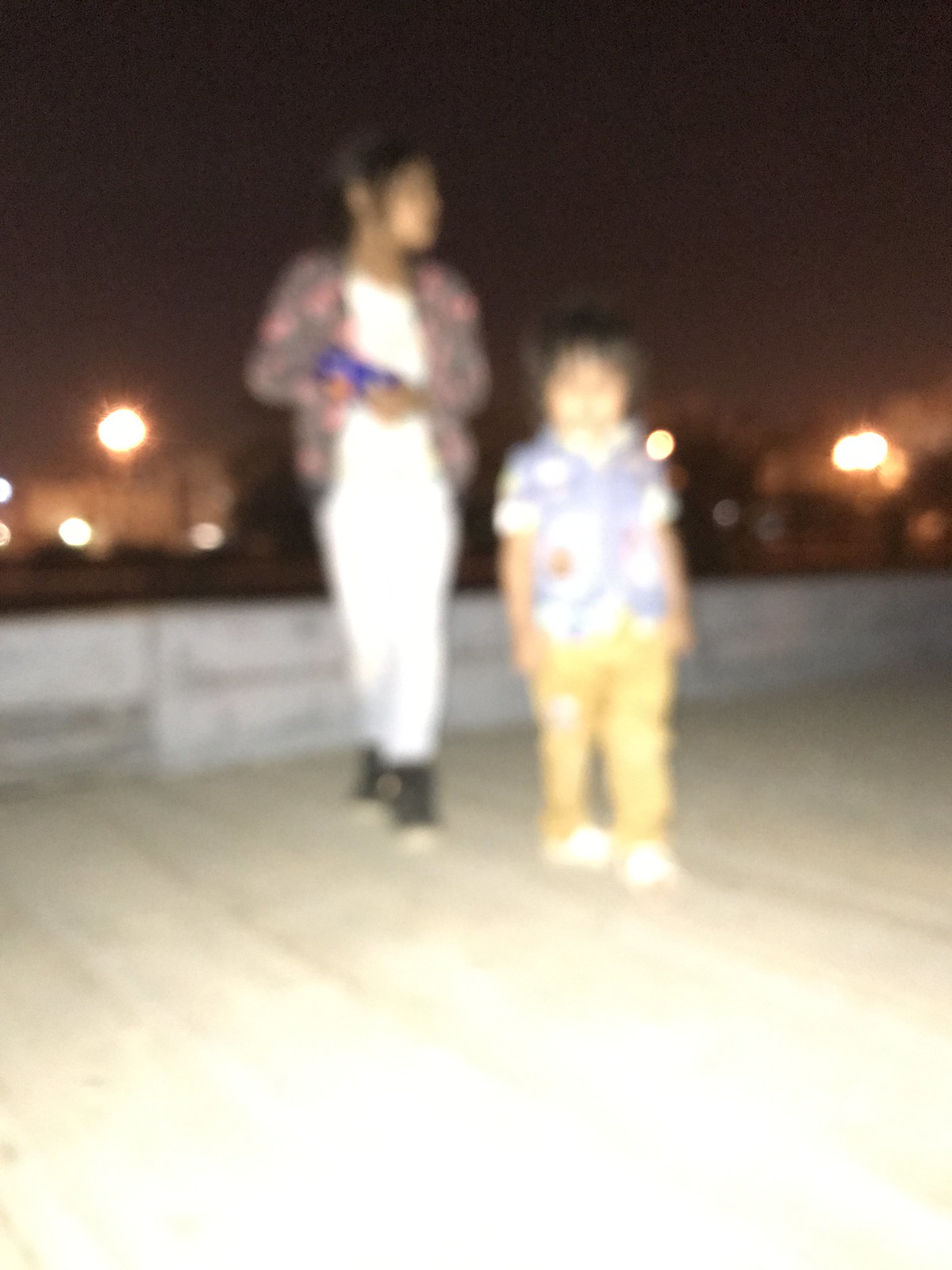In this blurry photo, two children stand eye level with the camera on what appears to be a wooden dock with a grayish half wall behind them, illuminated by distant orange and pink lights that dot the darkened sky. The child on the right, who sports brown pants, white shoes, and a blue shirt, has dark hair in a short bob cut and gazes directly at the camera. The older, taller child on the left wears white pants, black shoes, a white shirt, and a red and black overshirt; they hold something blue in their hand and look off to the left. The wood beneath them is a tannish white. Overall, the scene is dimly lit, suggesting the sun has already set, accentuating the serene night ambiance.